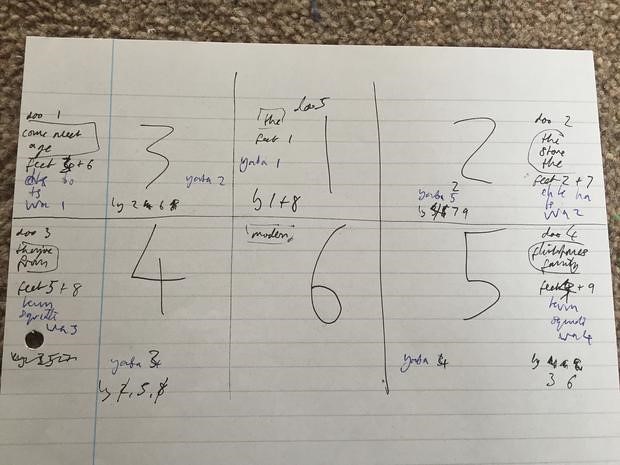This indoor color photograph captures an overhead view of the upper portion of a piece of white notebook paper adorned with horizontal lines. The paper, positioned on a low-pile brown carpet that is visible in the upper left and right corners, features several hand-drawn numbers using a pen. 

The paper is divided into a grid by one horizontal and two vertical lines, creating three columns and two rows. In the upper left cell of the grid, the number "3" is written, followed by "1" in the center cell and "2" in the rightmost cell of the first row. The second row contains the numbers "4" in the left cell, "6" in the center, and "5" in the right cell. 

Additionally, the paper contains some illegible scribbles in both black and blue pen along the left and right margins, suggesting perhaps an attempt at mathematical doodling or solving a puzzle. Some faint, nearly illegible numbers are also discernible at the bottom left of each grid cell. Despite their lack of clarity, the photograph is well-lit and sharply focused, offering a clear view of these elements.